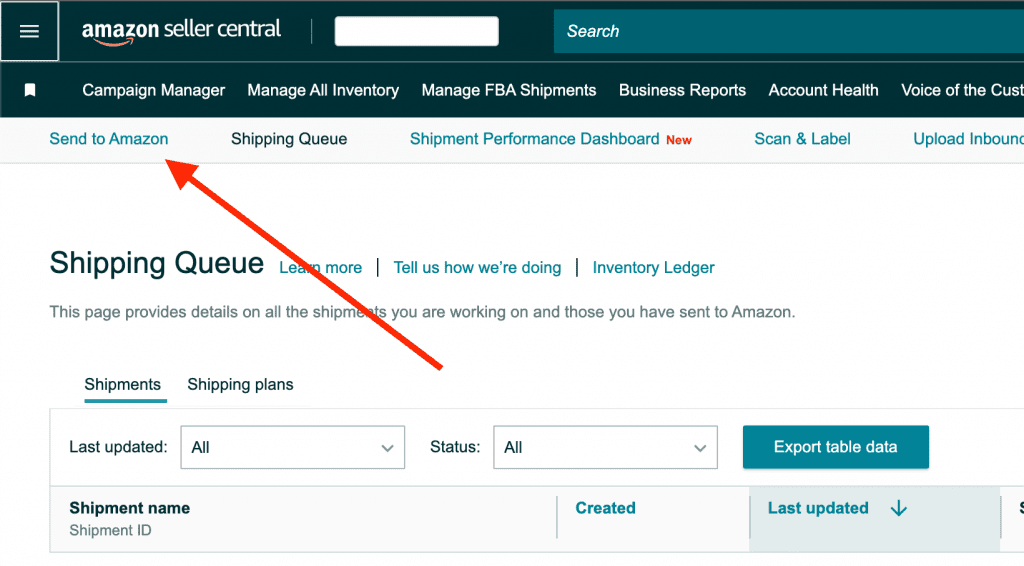This image is a detailed screenshot of the Amazon Seller Central dashboard, tailored for businesses and individual sellers managing their Amazon operations. 

In the top left corner of the interface, there is a recognizable hamburger menu icon, consisting of three horizontal stripes on a bluish-green background, which likely leads to settings and other navigation options. Beside this, the text "Amazon Seller Central" is prominently displayed.

On the far right of the top navigation bar, there is a search tab to facilitate finding specific information or tools within the platform.

Directly below the top navigation, there is a dark green menu bar with white text, offering various operational tabs: 
- Campaign Manager
- Manage All Inventory
- Manage FBA Shipments
- Business Reports
- Account Health
- Voice of the Customer

An eye-catching red arrow points to the first tab below this main menu, labeled "Send to Amazon," which directs users to the shipments form below. Adjacent to this, tabs include "Shipping Queue," "Ship Performance Dashboard" (marked as "New" in red text), "Scan and Label," "Upload Inbound," and another "Shipping Queue." Below these tabs, additional options read "Learn More," "Tell Us How We Are Doing," and "Inventory Ledger."

The detailed central section of the page gives a comprehensive view of all shipments being processed or sent to Amazon. Here, users can find and manage shipment information based on various criteria. The "Shipments" tab is active, showing categories such as "All Status," "All Export Table Data," with fields for "Shipment Name," "Shipment ID," and timestamps for when items were "Created" and "Last Updated." Currently, no specific shipment details have been filled in.